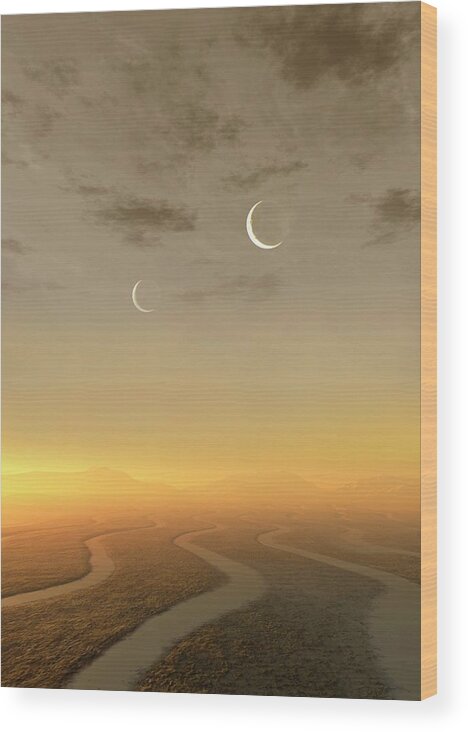This artwork, printed directly onto a wooden canvas that is slightly tilted to the left, presents a vivid and detailed scene of an otherworldly landscape. The painting features three equidistant rivers flowing through lush, well-maintained grasslands, which could also be interpreted as dense forests. Above these rivers, the tranquil sky captures attention with two small crescent moons that suggest the scene might be on an unearthly planet. The sky transitions from a cloudy gray at the top to shades of orange and yellow near the horizon, indicating a sunset. There are also wispy, dark gray clouds adding texture to the upper part of the image. Sunlight beams down softly, introducing hints of pink and orange into the scene. The entire composition is set against a clear and spacious sky, conjuring both a sense of tranquility and mystery.